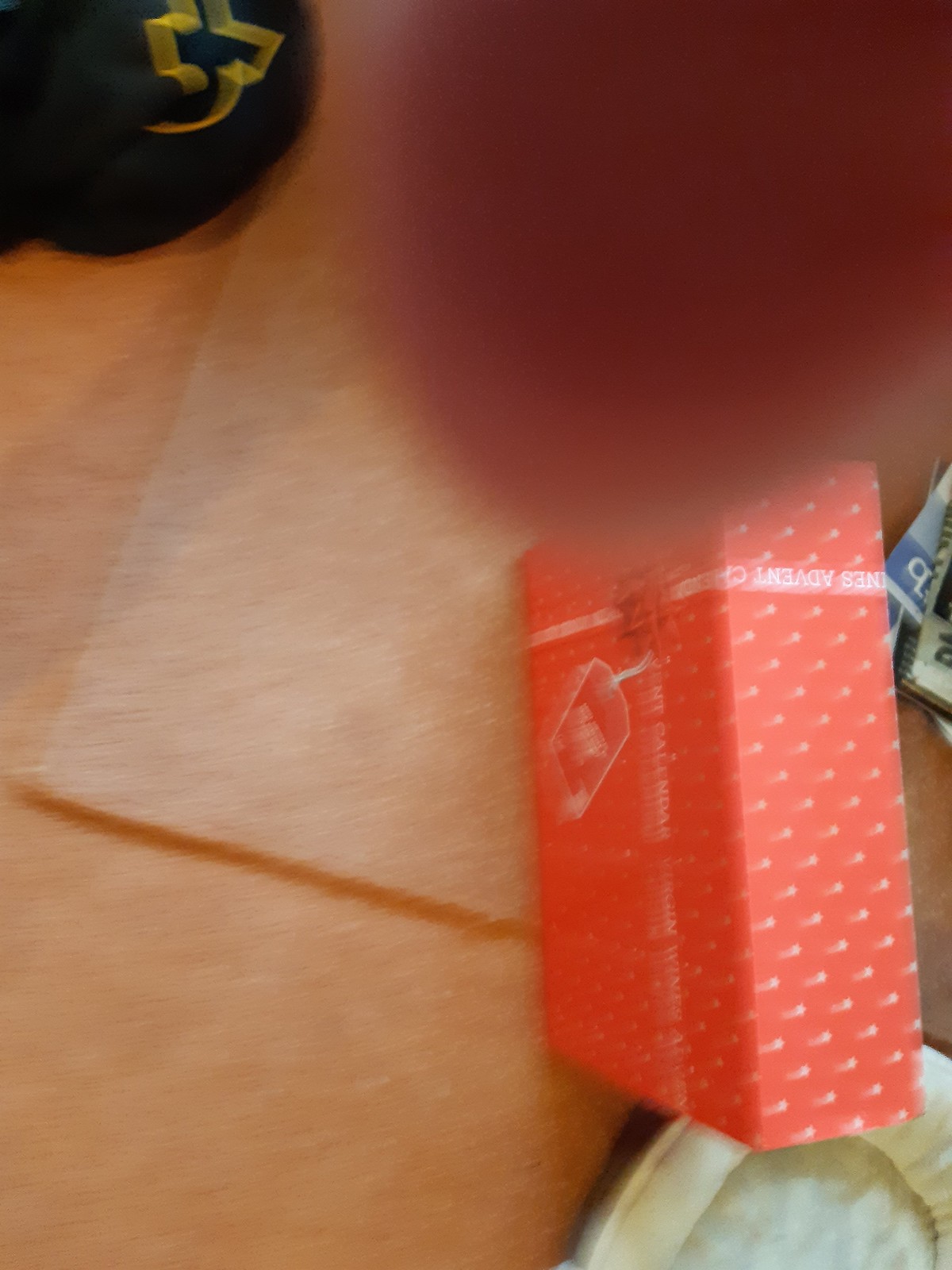A small, red box adorned with white polka dots is situated on a tiled floor featuring rust-colored grout. The box, which is upside down and displays some white writing, appears slightly out of place. Behind the box, a black hat with gold lettering is partially visible. A blurry, reddish object that seems to resemble a thumb or finger is also present in the image, adding a touch of intrigue. Additionally, there is a pile of magazines or possibly a pet bed in the background, enhancing the scene's eclectic nature.